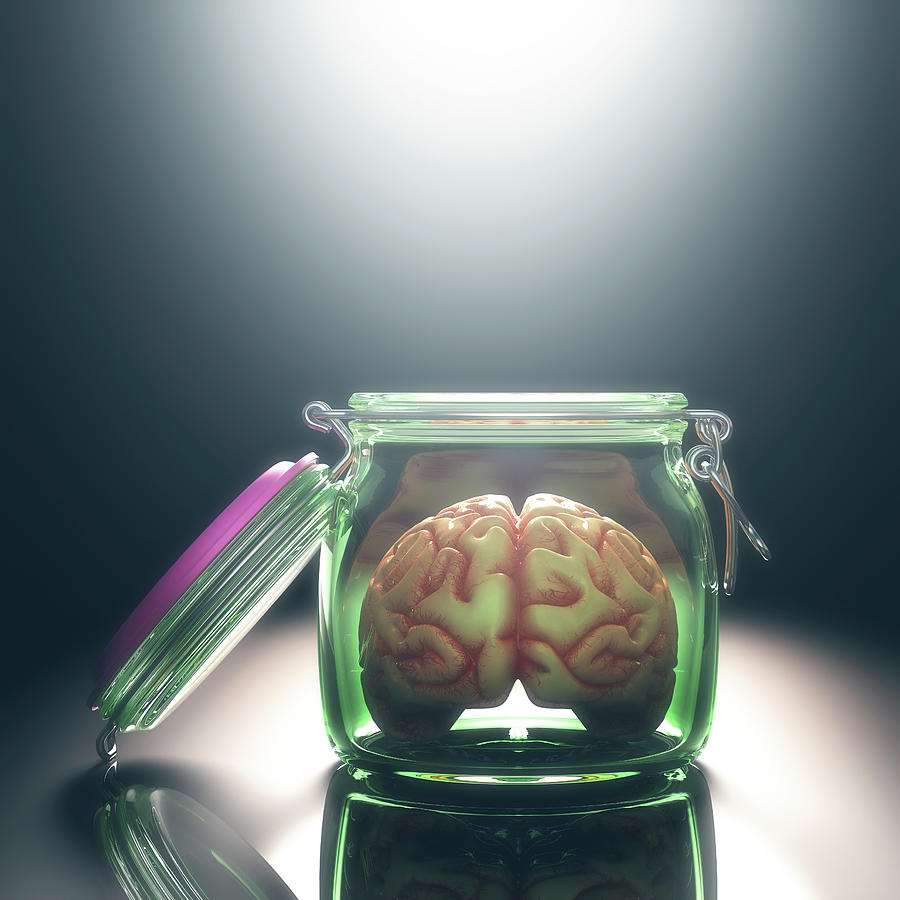The image showcases a highly detailed photograph of a translucent glass jar with a pink rubber stopper lid, placed on a sleek, reflective, mirror-like surface that captures the jar and lid's reflections vividly. Inside the jar, there's a replica of a human brain, characterized by its realistic ivory color and intricate red grooves. The jar has a subtle green tint along its edges, adding a unique hue to the display. Above, the background transitions to a dark gray shade, culminating in a very bright light at the top center, illuminating the scene with dramatic effect.